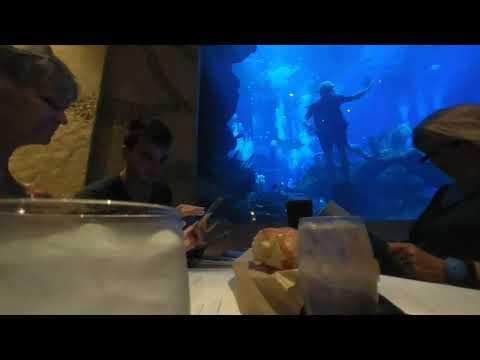The image depicts a group of people seated at a table in a restaurant that appears to be situated within an aquarium. The scene is viewed from a camera placed on a table, with a cup containing ice in the bottom left corner. In the immediate foreground, glasses of water and possibly a bread basket are visible. At the center of the image, three people, including a younger Caucasian man and two older white women, are gathered around the table, seemingly engrossed in reading menus or looking at their cell phones.

Dominating the background is a large aquarium, taking up nearly the entire wall. The vivid blue hue of the aquarium stands out and serves as the backdrop for the dining experience. Inside the aquarium, a diver can be seen swimming near the glass, gesturing to the right. The setting is undeniably indoors, though the time of day is indeterminate. The color palette of the image includes black, various shades of blue, brown, tan, white, and silver, providing a rich visual contrast. Notably, there is no text visible anywhere in the image.